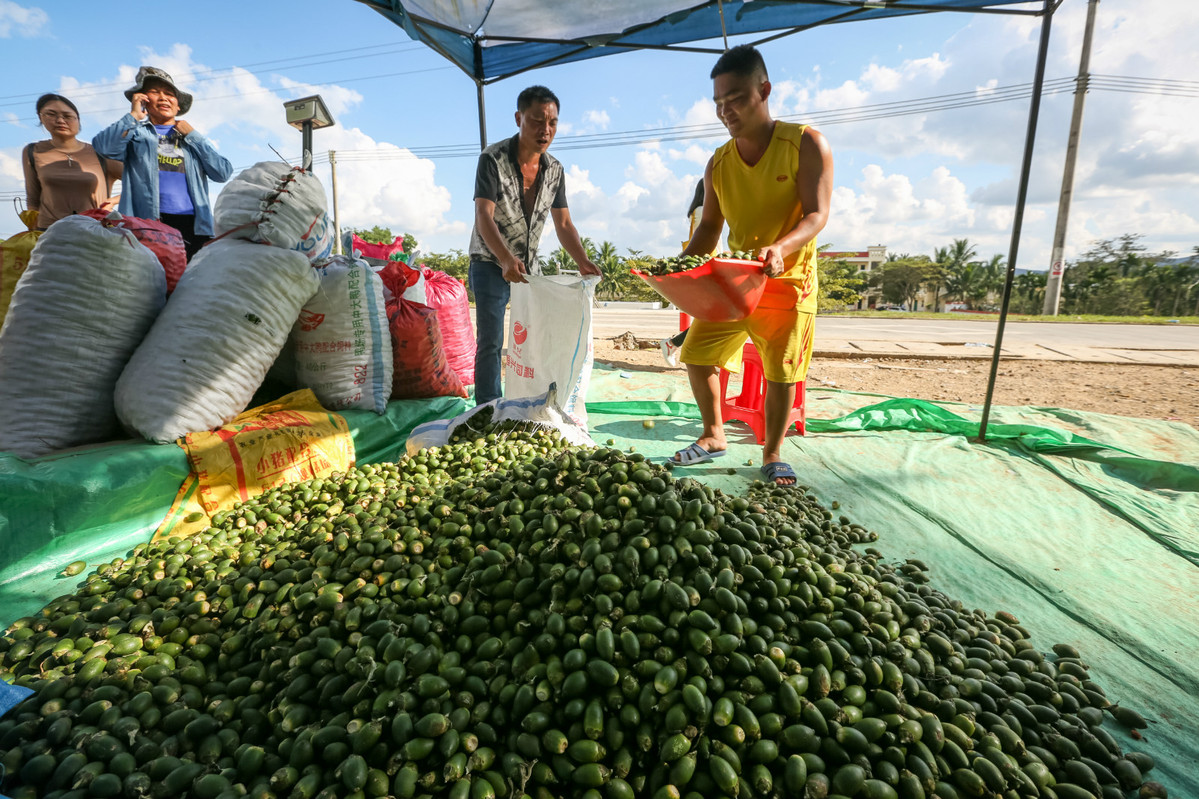In this vibrant outdoor photograph, four people, presumably farmers, are engaged in the harvesting and bagging process of a green, oblong-shaped fruit or vegetable that is about the size of an adult's palm. The scene is set beneath a pop-up tent that provides shade as they work. At the center of the image, two men are actively bagging the harvest. One man is holding a large open white sack, while the other man holds a red plastic bucket filled with these mysterious green produce items, possibly about to pour them into the sack. A substantial pile of these green fruits or vegetables lies atop a green tarp spread on the ground, extending from the foreground to the middle of the photograph.

In the upper left corner, a man and a woman stand near a series of colorful bags—white, red, and yellow in hue—indicating that these are the filled sacks of the harvested produce. Some bagged items can also be seen neatly stacked in the background. This backdrop includes what appears to be the field or seeding area from where the produce was harvested. The four individuals, all appearing to be of Asian descent, diligently perform their tasks under the awning, contributing to what seems to be a communal effort to prepare the harvest for the market.